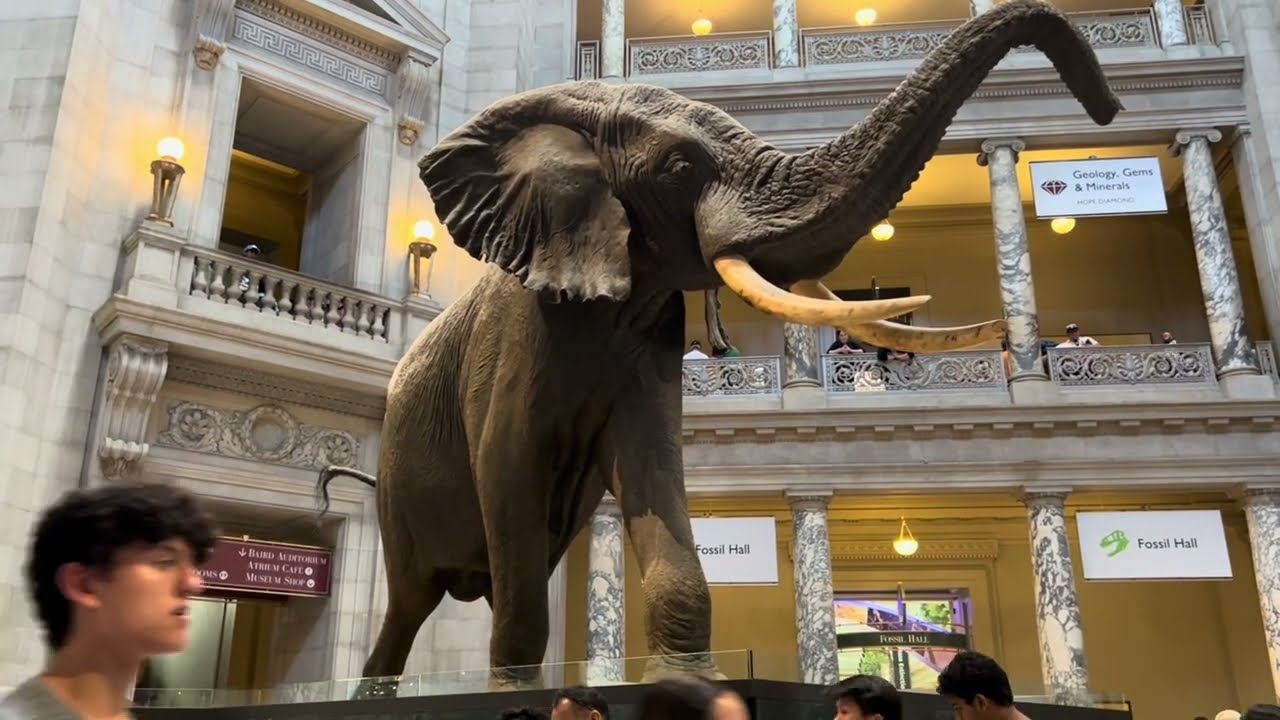The image captures the grand interior of a spacious, multi-level foyer within a science museum or university building. Dominating the scene is an impressively detailed elephant statue, facing right with its ears flared, tusks protruding, and trunk extended. The statue is mounted on a raised pedestal, highlighting its immense size relative to the people milling about the foreground. Among these individuals, a young man with dark, curly hair stands out on the left. The building itself exudes a mid-century regal charm, characterized by ornate stone columns reminiscent of Roman architecture, and multiple levels with visible etched details. Hanging signs provide direction within the hall, including one that reads "Fossil Hall." The photograph, taken in landscape orientation, encapsulates a sense of educational grandeur and timeless elegance.